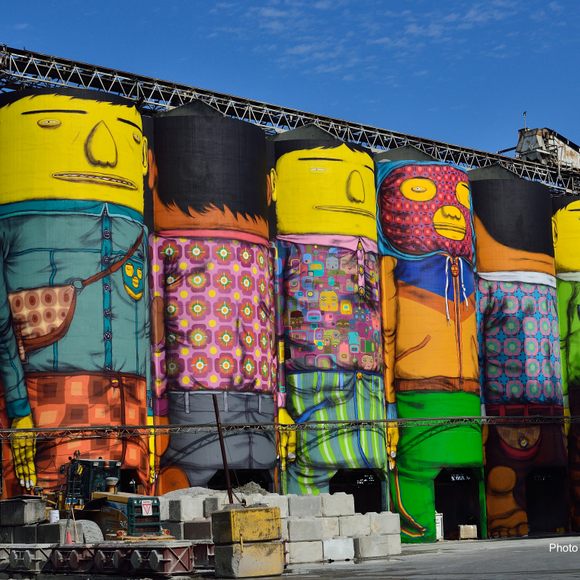The close-up photograph showcases an eclectic collection of seven cylindrical inflatables designed to resemble cartoon-like individuals, seemingly part of an artistic installation in an industrial area. Each figure has a yellow face and black hair, with detailed and colorful attire that contributes to the vibrant and whimsical aesthetic.

The first character wears a blue shirt with a matching blue pocket, a round purse with circular patterns, and a brown and orange plaid skirt, accessorized with yellow hands. The next figure stands with its back to the camera, displaying an orange-colored skin and a pink shirt adorned with pink, purple, and red flower-like circles, some centered with yellow or red, paired with gray pants.

Facing us, the third figure showcases a multicolored shirt featuring blocks of yellow, purple, blue, red, and green, alongside green, white, and blue striped plaid pants. Another character is distinct with a blue hood, a red face mask with smaller red circles and yellow interiors, and an orange sweater with a dark blue spot on the hood, paired with light green pants.

One of the figures, presenting a back view, wears a blue patterned shirt with red circles, green centers, and dark green outlines. The last visible individual is cut off, revealing just a light green sweatshirt. The inflatables stand amidst a setting lined with gray and beige bricks against a gray concrete surface, under a cyan midday sky with an industrial gray bridge or scaffolding above, possibly traversed by a train. The scene blends creative art with an industrial backdrop, creating a surreal and slightly eerie visual experience.